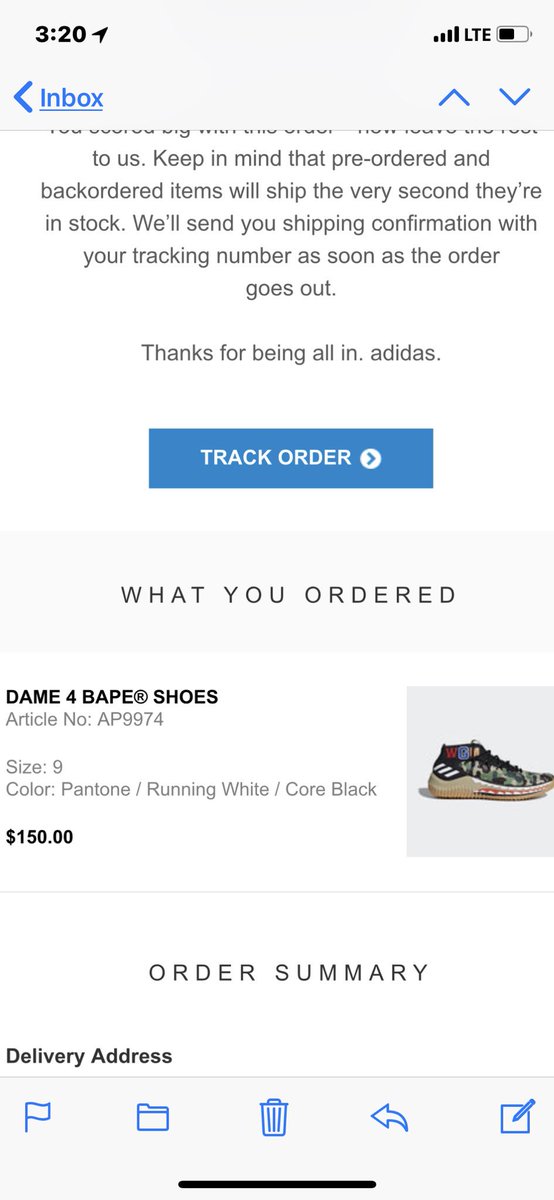In this image, we see a detailed screenshot of a web page on a mobile device, indicating an order confirmation. At the top of the screen, system indicators show "3:20" in black numbers, "LTE" network status, signal strength bars, and a battery icon that is approximately half-full. 

On the left side of the screen, "Inbox" is displayed in blue with a left-pointing arrow, suggesting the user is in their email application. Next to this, an up-and-down arrow icon is visible. Below this header, there is a partially visible message from Adidas, which reads: "Keep in mind that pre-ordered and back-ordered items will ship the very second they're in stock. We'll send you shipping confirmation with your tracking number as soon as the order goes out. Thanks for being all in, Adidas. "

Further down, there is a blue rectangular button labeled "Track Order." Beneath this, the section titled "What you ordered" specifies that the user has purchased a pair of Dame 4 BAPE shoes in size 9 and color combination Pantone running white and core black. To the right, an image of the shoes is displayed. The price of the pair is listed as $150.

An "Order Summary" heading is visible next, but the details beneath it are obscured. At the bottom of the screen, there are icons for a trash can, an arrow, a note-taking option, a folder, and a flag. The final section displays a headline for "Delivery address," though the specifics are not visible. The overall layout and context hint at the user reviewing their online purchase details via a mobile email confirmation.